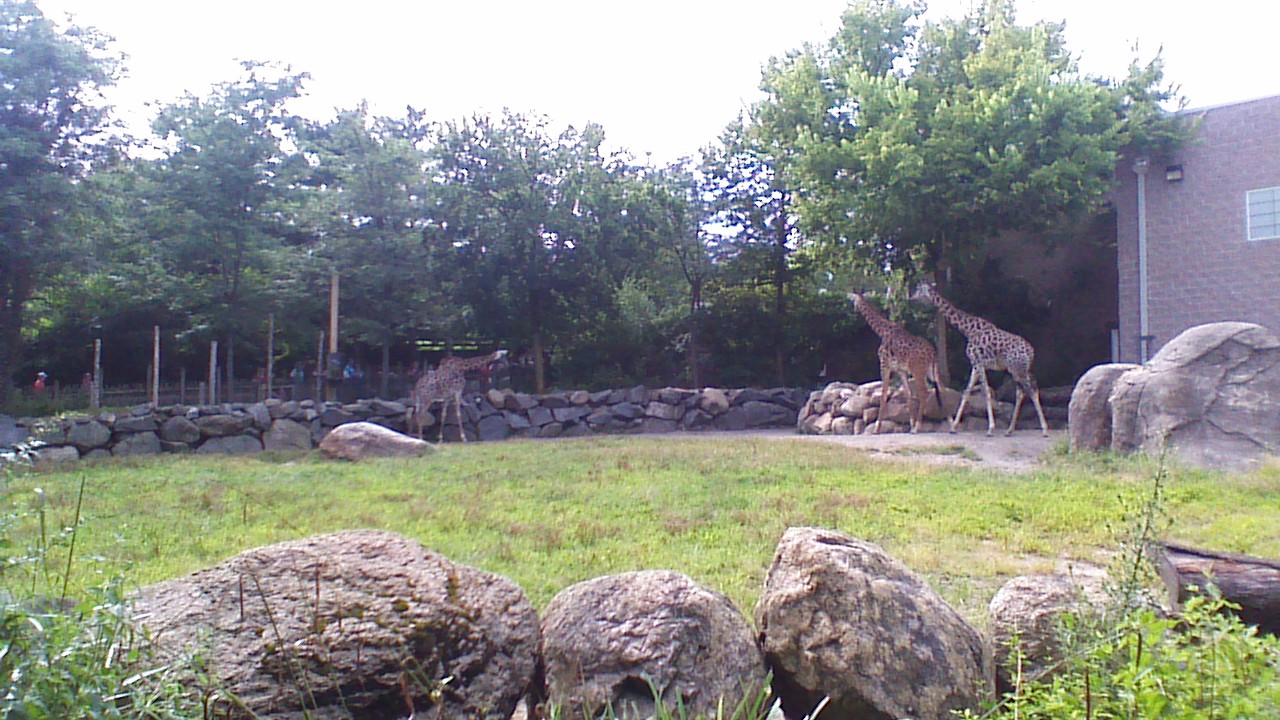In this real-life outdoor photograph of a zoo enclosure, three giraffes are the main focus. Two giraffes are on the right side, craning their necks to munch on the thick, full green leaves of a tree, while the third giraffe stands slightly left of center, gazing out at the crowd of onlookers surrounding the enclosure. Inside the enclosure, the ground is covered in thick, green grass and adorned with several large, decorative boulders and rocks that form a low, circular stone wall. Behind this wall, a walking trail allows zoo patrons to observe the exhibit. Adding to the scene, a log is visible on the ground, and a brick building with an orangey-brown hue stands near the large tree. The building features a small window, an opening likely used for the giraffes’ nighttime shelter, and a light pole. The entire exhibit is surrounded by lush, green trees under a gray sky, with the crowd of people watching the enchanting giraffes from behind fencing.